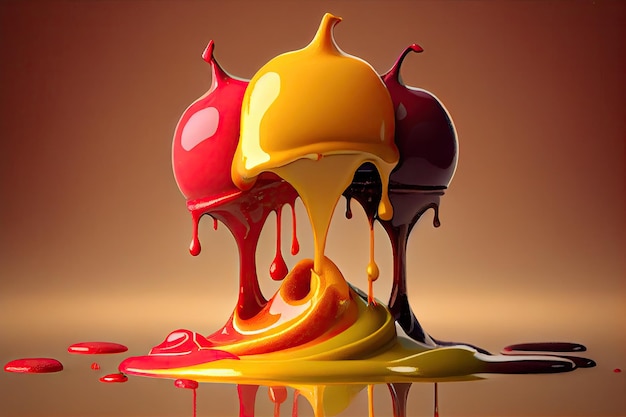The image features three large, shiny, candy-like objects resembling Hershey's Kisses or dipped cherries, hovering against a goldish-brown background. Each object is a different color—bright red, yellow, and a deep crimson-brown. They appear to be dripping paint, with vibrant, viscous trails spilling onto the ground beneath them. This dripping paint forms swirling mounds of mixed colors on the surface below, creating distinct and vibrant patterns where red, yellow, and brown merge slightly but largely retain their own hues. The objects have stems, further enhancing their resemblance to dipped cherries or other fruit, and the entire scene emanates a surreal, vibrant, and artistic quality.